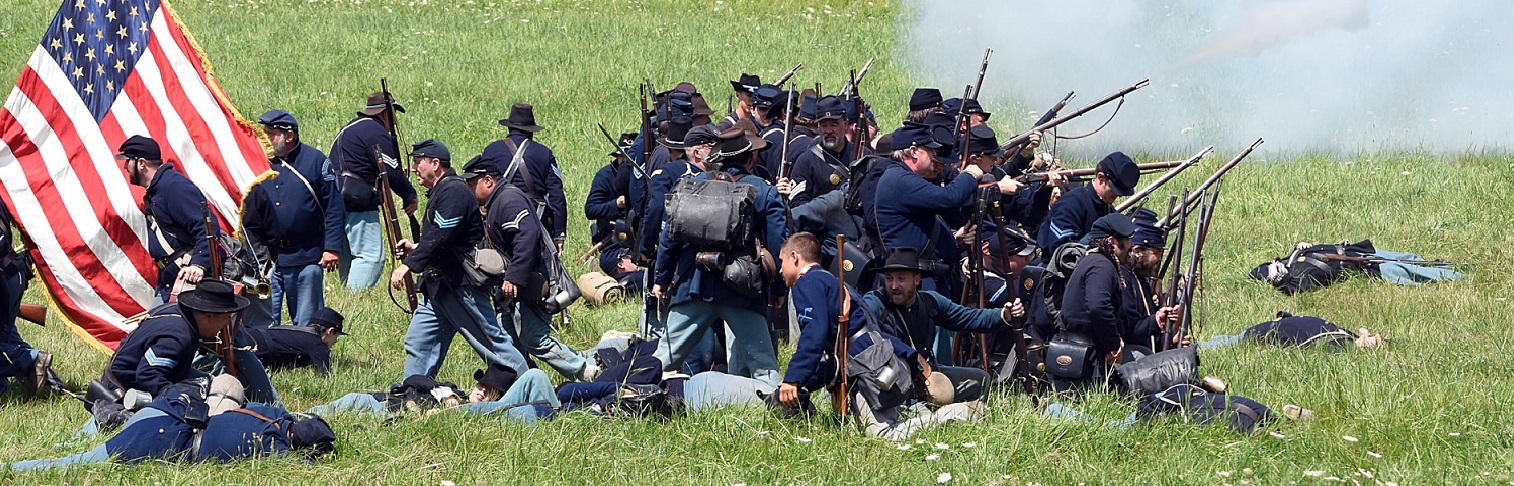This is a panoramic photograph capturing a vivid Civil War reenactment. The scene is dominated by a large group of soldiers clothed in Union uniforms—dark blue caps, coats, and blue jeans—spread across a field. Many soldiers are depicted firing their muskets, creating a dense cloud of smoke that drifts into the air, primarily on the right-hand side of the image. Among the standing soldiers, several are pointing their rifles both upward and outward into the distance, simulating a battle stance.

Scattered throughout the field, a number of reenactors lie on the ground, portraying slain or injured soldiers. Notably, on the right side of the image, there are three such men isolated from the main group. In the center, the density of soldiers is highest, with the action flanked by both fallen and retreating figures. Leading from the left, an individual carries a large, historically accurate American flag with fewer stars than the modern version.

This detailed snapshot seems to depict a segment of a Civil War retreat, with some soldiers staying behind to provide cover fire as others fall back, underscoring the chaotic yet organized nature of historical warfare.